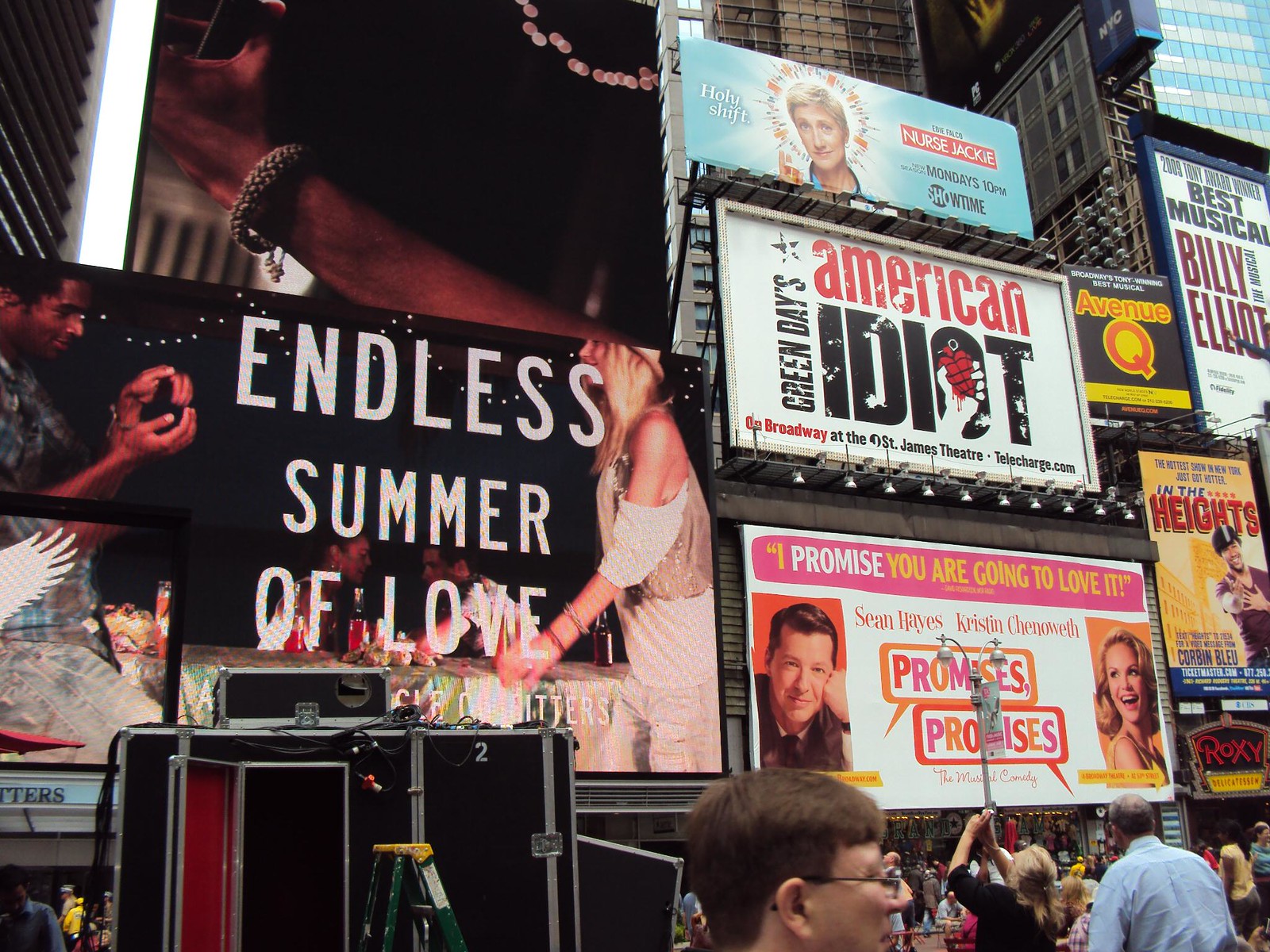In the bustling streets of a metropolitan city, people stand on the sidewalk or street, gazing upward at a towering array of vibrant billboards attached to the sides of skyscrapers. To the right, three billboards are stacked vertically. At the top, in bold white letters, it proclaims "Nurse Jackie," featuring a woman with short blonde hair, with the phrase "Holy Shift" and the showtime "Mondays at 10 p.m. on Showtime" in red and white lettering. Below it, another billboard promotes "Green Day's American Idiot" on Broadway at the St. James Theater, with the text displayed sideways up the left side. The bottom billboard quotes, "I promise you are going to love it," endorsing the musical "Promises, Promises" starring Sean Hayes and Kristin Chenoweth, with their photos on either side. On the left-hand side of the image, another prominent billboard reads "Endless Summer of Love" in white letters against a black background. Amidst these main attractions, additional signs for popular shows like "In the Heights," "Avenue Q," and "Billy Elliot" add to the vibrant tapestry of advertisements. The scene is peppered with city dwellers, some capturing the moment with their cameras, others immersed in the urban ambiance, a man in a blue Oxford shirt among them, heads tilted upward to take in the colorful spectacle.